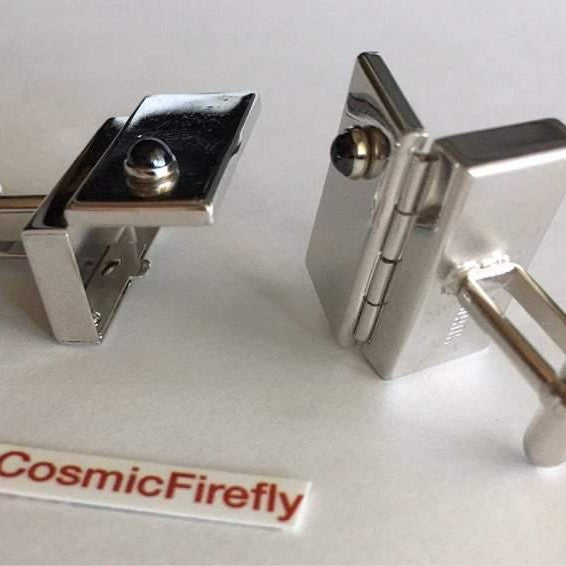This close-up photo features two chrome or silver metallic objects, likely cufflinks, resting on a white surface. Each item has a box-shaped enclosure with a hinged lid that opens. The left cufflink is open, revealing an empty compartment, while the right cufflink shows the mechanism where it would pass through buttonholes. Both cufflinks are adorned with a dark, round gem on the side of the top of each lid, encircled by a silver band. Notably, one cufflink lies horizontally with its hinge open, and the other stands vertically like a book on a shelf, its hinge also flipped open. These objects are positioned in such a way that highlights their intricate design and functionality. In the bottom left corner of the image, there is a white label with red text from a label maker, reading "CosmicFirefly" without a space between the words.